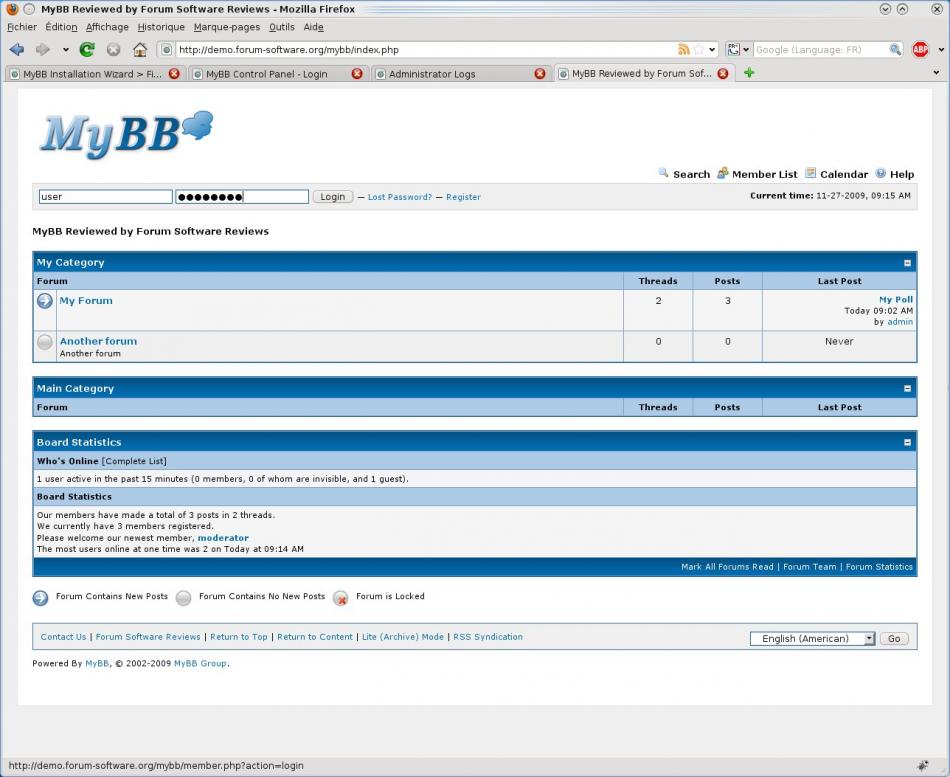This is a detailed screenshot of a Firefox browser window displaying a review of the forum software MyBB by Forum Software Reviews. The browser tab's title reads "MyBB Reviewed by Forum Software Reviews - Mozilla Firefox." 

The interface of the forum demo has a gray background complemented by white sections and accented with dark and light blue hues. In the top-left corner of the forum, the MyBB logo is prominently displayed, featuring overlapping chat bubble icons with a gradient of light to dark blue.

A login box is visible, prefilled with the username "user," while the password field is obscured by black dots. The forum showcases sample categories including "My Category," "Main Category," and "Board Statistics." Within "My Category," there are two sample forums: "My Forum" and another unnamed forum, providing a demonstration of the forum structure with minimal content. "My Forum" contains 2 threads and 3 posts, while the "Main Category" is currently empty, containing no forums.

The "Board Statistics" section provides real-time information about forum activity. It shows that one user has been active in the past 15 minutes, which includes zero members, zero invisible users, and one guest. The statistics also indicate a total of 3 posts made in 2 threads, with 3 members registered. The newest member is named "moderator." The record for the most users online simultaneously is 2, achieved today at 9:14 AM.